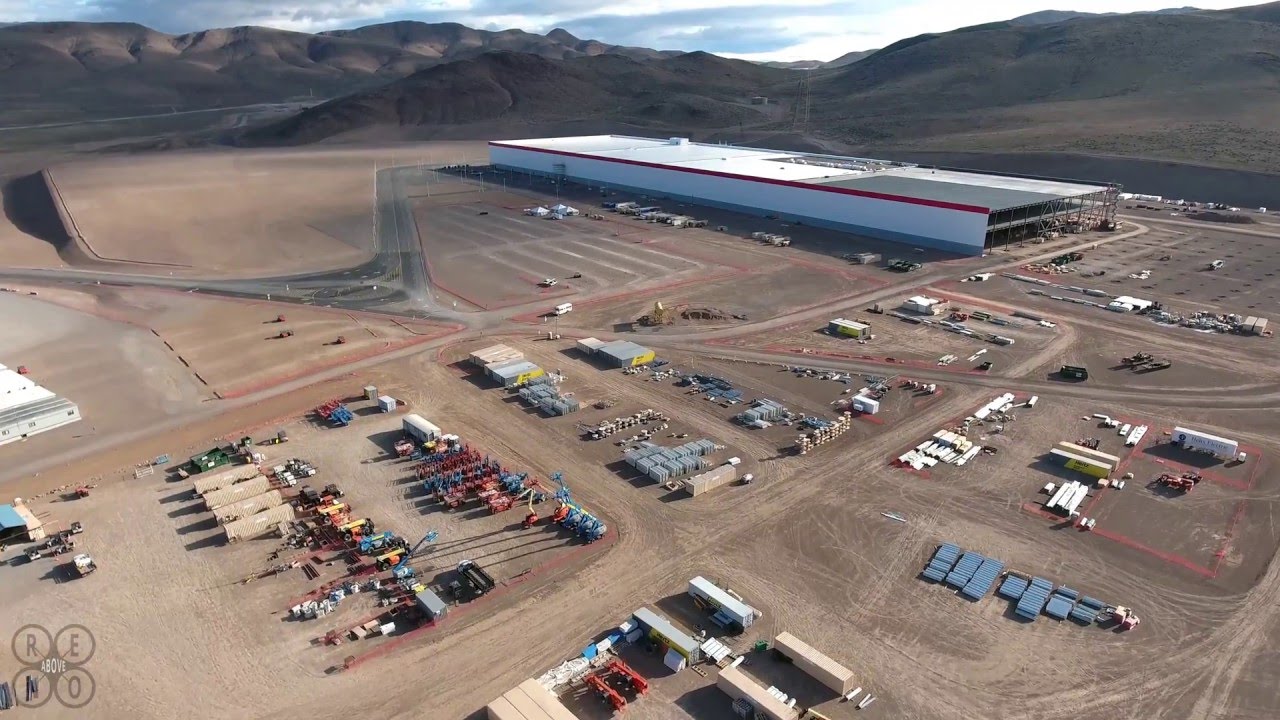The aerial image showcases a daytime view of an expansive outdoor area, featuring a diverse arrangement of buildings and structures spread across a brownish-gray dirt landscape. In the far distance, a picturesque blue sky with feathery white clouds rests above a rugged grayish-black mountain range. The most prominent structure is a long, rectangular building, white with a red stripe at the top and a gray or blue stripe at the bottom, located towards the middle to top-right part of the image. This building resembles an airport hangar and is adjacent to a nearby runway, though no planes are visible.

The scene is divided into distinct sections by numerous dirt roads and small streets, with various rectangular buildings of different colors scattered throughout. Vehicles are parked around these buildings, with long trailer-like structures adding to the complexity of the layout. On the flat roof of the main building, there seems to be an open area with metal bars, giving it an industrial look.

In the bottom left-hand corner, four circles spell out "R-E-N-O." These circles are small but distinct, adding a unique identifier to the image. The overall composition of the image, from the expanse of dirt roads and buildings to the distant mountains and sky, offers a detailed snapshot of this intriguing and structured landscape.